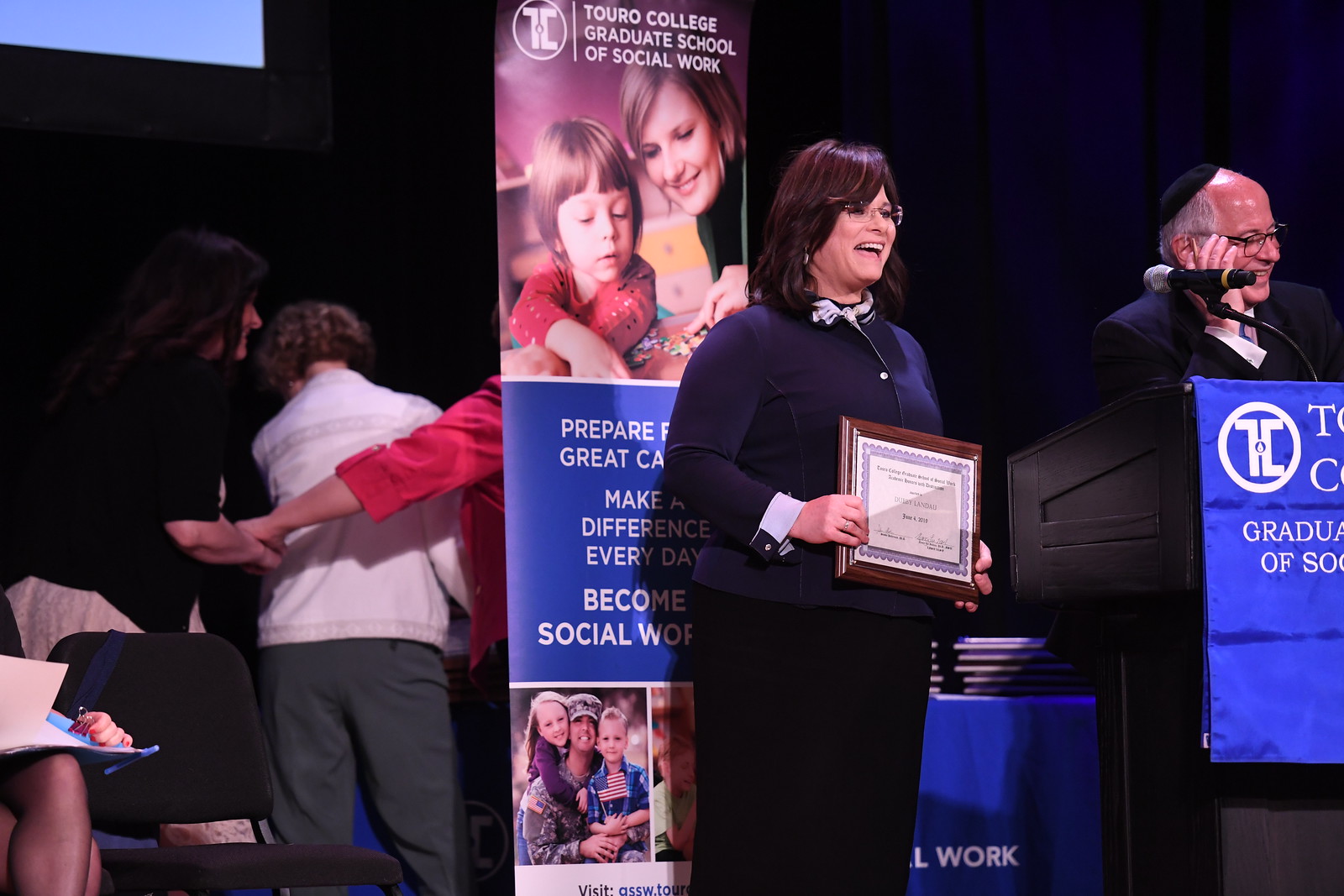The image captures a jubilant woman standing on a stage, holding a framed plaque or diploma in both hands. She is dressed in a dark blue long-sleeve shirt and a long black skirt, and her shoulder-length brown hair features subtle highlights. She wears glasses and displays a wide, open-mouthed smile. To her right stands an older man behind a black podium adorned with blue drapery and partially visible white letters. The man, who is smiling, has gray hair, is balding with a shiny forehead, and wears glasses and a yarmulke. The backdrop features multiple banners labeled "Touro College Graduate School of Social Work," including an image of a woman and child working on a puzzle. To the left of the stage, three other people appear to be standing closely together, possibly embracing. Additionally, a blue table positioned behind the main subjects suggests the presence of other awards or diplomas, contributing to the celebratory atmosphere which hints at a graduation or awards ceremony.